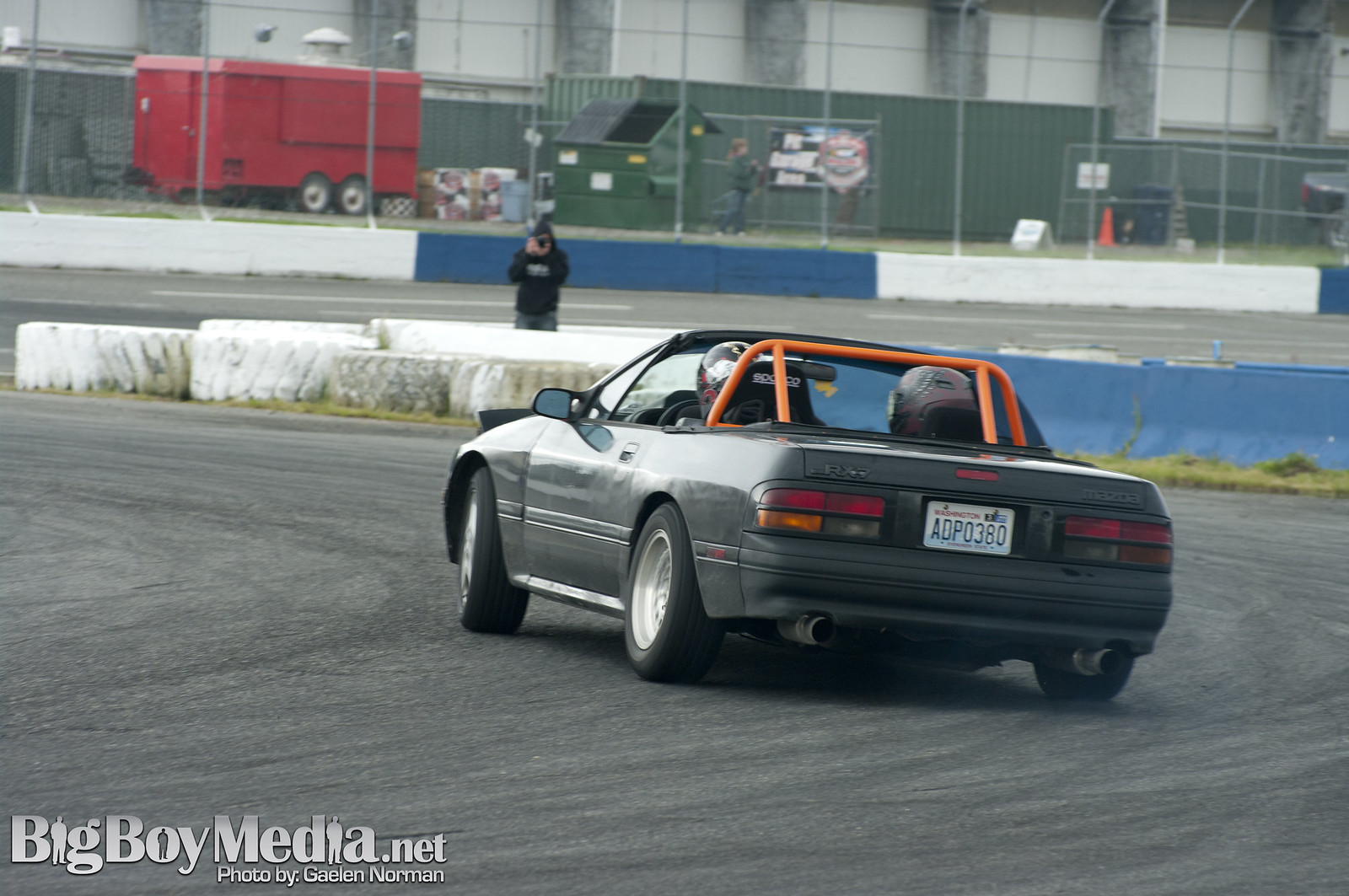This image showcases a dynamic scene of a matte black 1980s Mazda RX-7 convertible drifting around a corner on a closed racetrack. The car, which features distinct orange rollover bars and Sparco racing seats, is driven by a helmeted individual, with another person likely in the passenger seat. Emphasizing its custom look, even the Mazda emblems and the RX-7 logo are painted black. The car has a Washington license plate reading ADP 0380. On the other side of the curve, behind some protective white tires, a photographer captures the action. Additional elements in the background include a safety barrier, further parts of the racetrack, large buildings, a fence, and a dumpster. The scene includes colors like gray, light gray, brown, red, orange, blue, light blue, white, black, green, and different shades of gray. The lower left corner of the image is marked with the text "bigboymedia.net photo by Galen Norman."